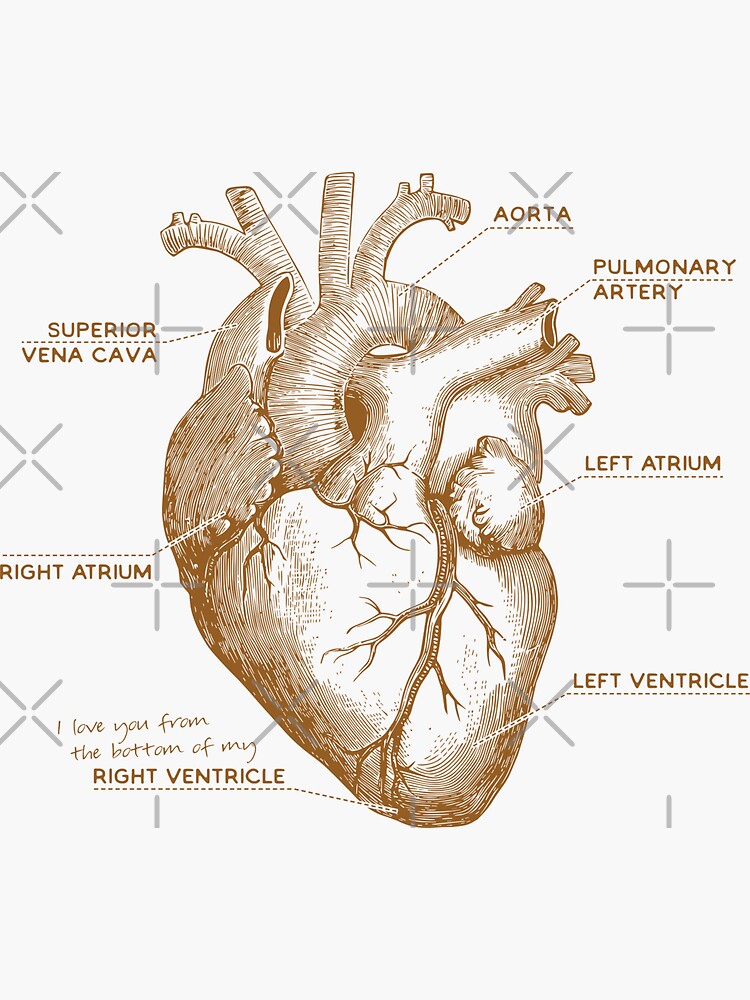This hand-drawn, detailed illustration of a human heart uses brown-colored lines and cross-hatching to add depth and texture. Labels identify various components, including the superior vena cava, right atrium, right ventricle, aorta, pulmonary artery, left atrium, and left ventricle. These parts are marked with small dotted lines connecting the text to the corresponding heart sections. The diagram also shows nerve-like structures and includes handwritten text near the right ventricle saying, "I love you from the bottom of my." Additionally, the image features semi-transparent, gray watermarks in the form of plus and x symbols. The overall background is light gray, enhancing the visibility of both the illustration and the watermarks.